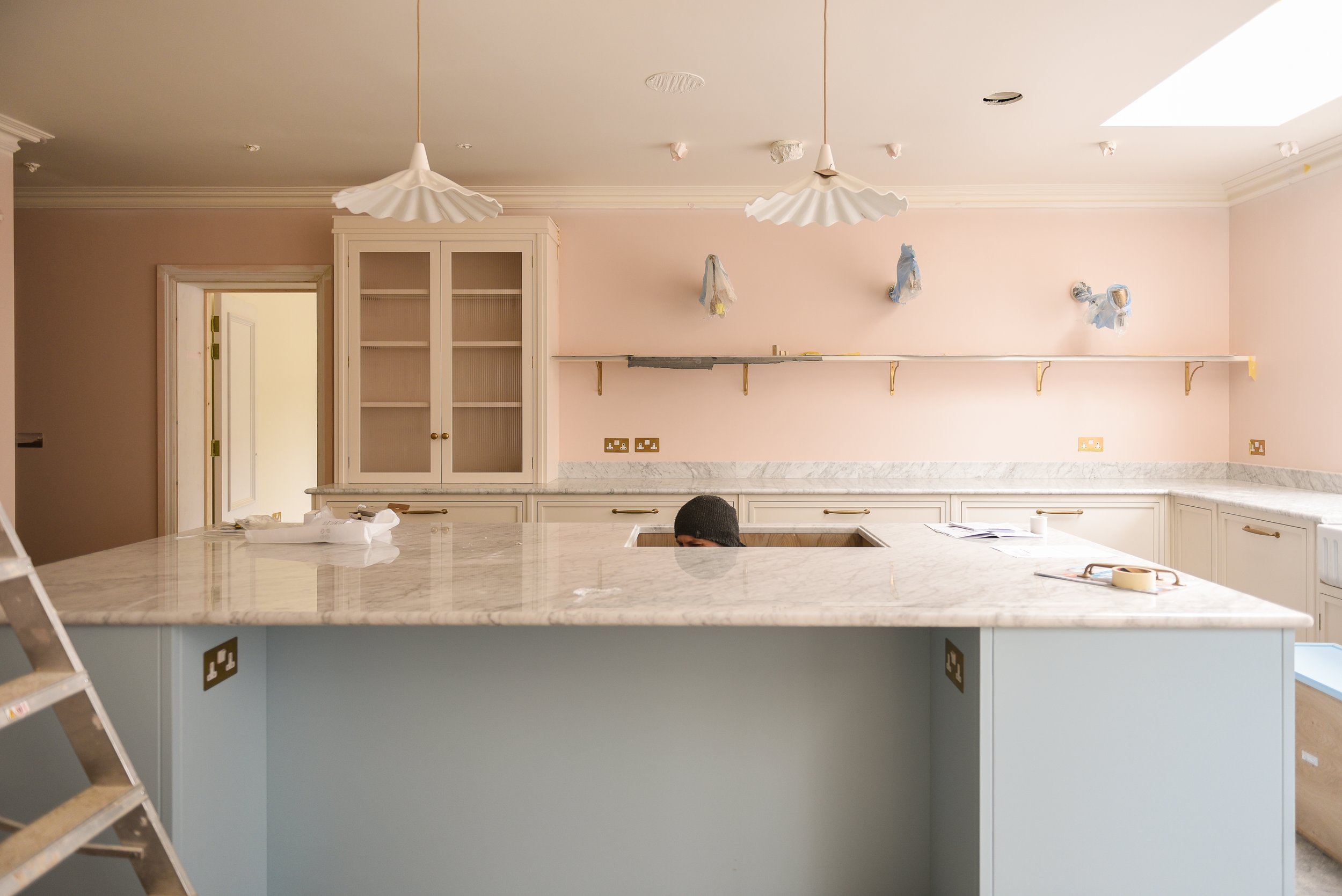This image depicts a large kitchen undergoing a remodel or new installation, characterized by its pristine white decor and pale peach walls. The countertop island, crafted from elegant white and gray marble, features a humorous yet unusual sight—a man's head poking through a hole where a sink is likely to be installed, with the man wearing a black hat. The foreground reveals a ladder positioned at the bottom left, while the countertop itself is cluttered with various tools, including scotch tape, manuals, and other construction materials. Electrical work appears in progress, with light fixtures yet to be installed, though one fixture is already mounted in the ceiling's top right corner. Shelving and cabinetry are partially constructed, enhancing the sense of an active workspace. The image suggests either preparation for a house sale or settling into a newly purchased home, portraying a blend of organization and chaos typical of a renovation project.